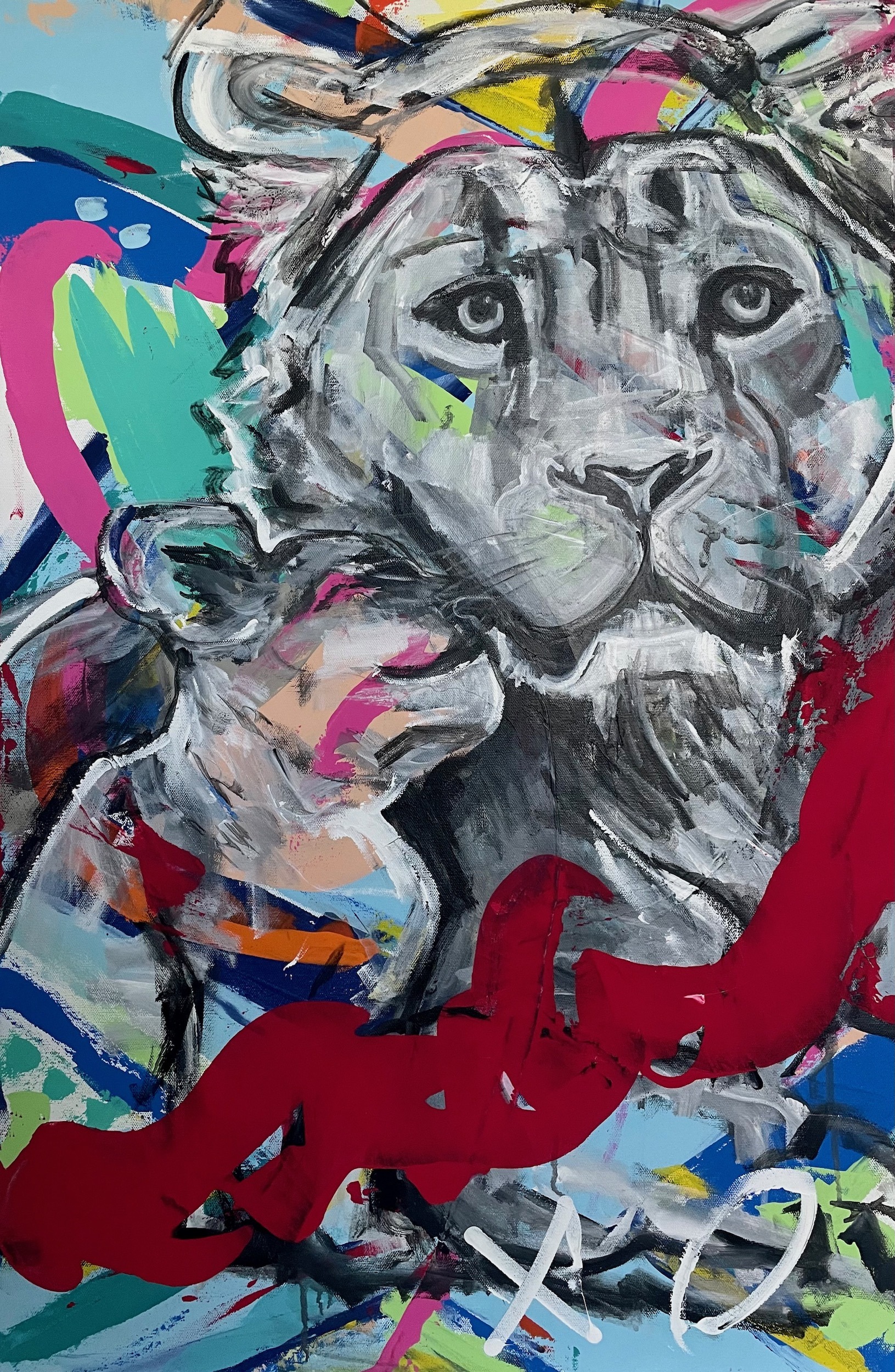The hand-painted artwork features a touching scene of a lion and its cub, rendered primarily in shades of black and white. The larger lion, positioned on the right, has a prominent head and gently nuzzles the smaller, left-leaning cub, whose eyes are closed in contentment. Accentuating this monochrome depiction are dynamic splashes of color—pink, blue, teal, orange, red, and beige—that streak through the lion's forehead and the cub's chest. The background is an abstract collage of vibrant brushstrokes and paint splatters, giving the piece a lively and somewhat chaotic atmosphere. At the bottom of the painting, a bold red streak stretches across the canvas, beneath which the artist's hand-painted signature "XO" appears in white. This expressive and colorful composition underscores the intimate bond between the majestic creatures.